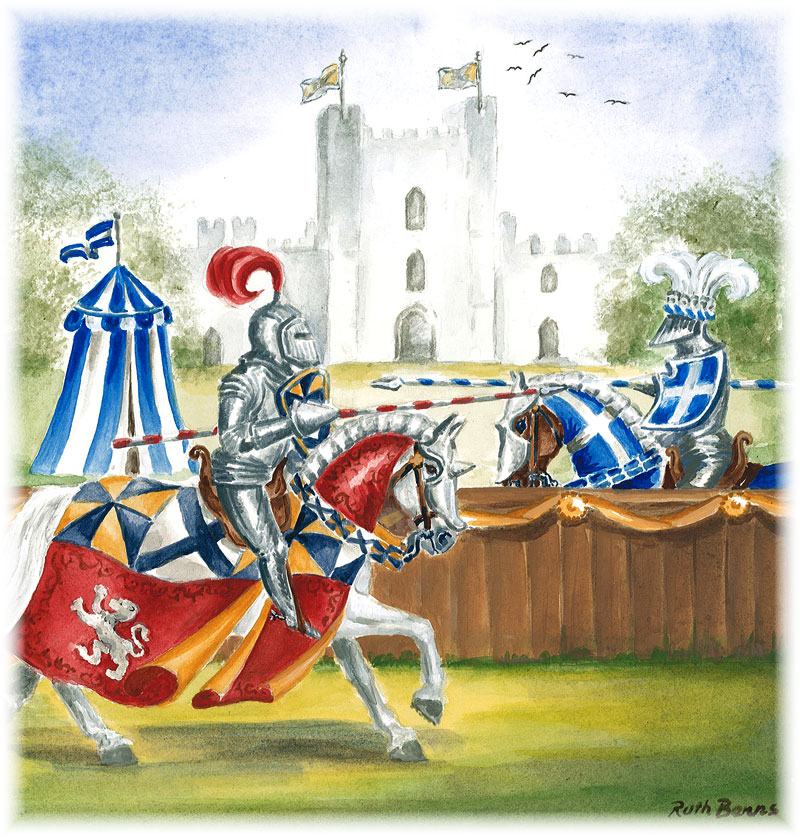In the foreground of this highly detailed painting by Ruth Burns, two armored knights are depicted jousting, each astride elaborately adorned horses. The knight on the left, riding a white horse draped in a vibrant red, blue, orange, and white cloth, holds a red and white striped lance. He is fully clad in silver armor with a striking red feather plume atop his helmet. His horse features intricate attire, including a silver lion emblem on the rear drape. His opponent, mounted on a brown horse covered in blue and white barding, brandishes a blue and white shield and a matching lance. This knight also sports a helmet with a distinctive white feather.

The scene is set against a backdrop of a grand medieval castle with a gray facade and two yellow-and-white flags fluttering from its main post. The sky is a serene blend of blue and white hues, with black birds soaring to the right of the castle wall. A blue and white striped tent, complete with a flag and situated to the left of the castle, further enhances the medieval ambiance. The ground beneath the jousting knights is a mix of green and yellow grass, casting gentle shadows. The entire scene is framed by lush green trees on either side and a brown wall adorned with ribbons, adding to the historical atmosphere. A wooden stage occupies the scene, adorned with the inscription "Roth beams on grass with a stage." At the bottom right corner, the artist's name, Ruth Burns, is signed in black.